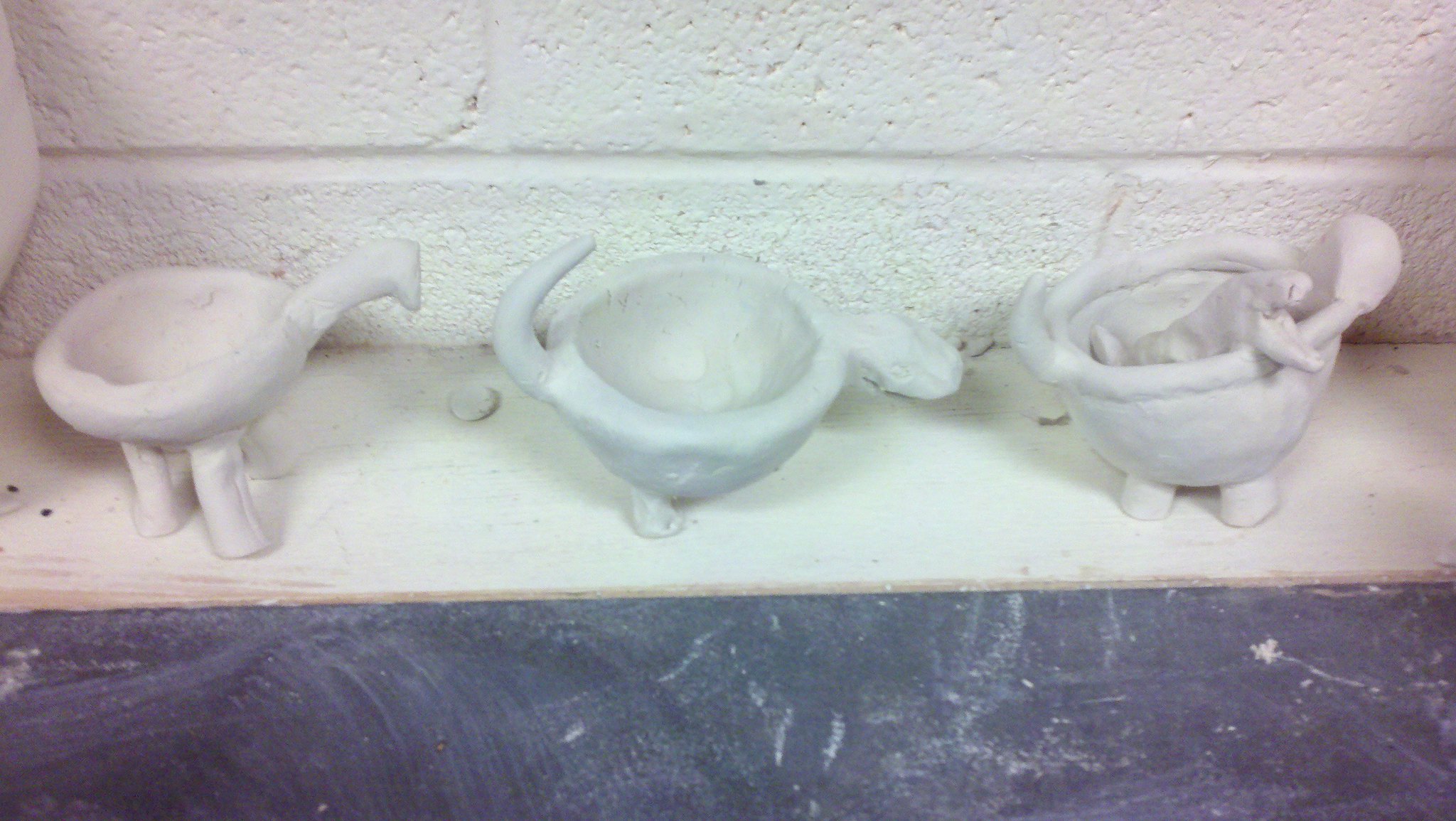This photo features three handmade ceramic or clay figures, seemingly in the early stages of creation, as they have not been kiln-fired or painted. Each figure has a bowl-shaped middle, indicating they might serve as containers, possibly for holding small items or kitchen sponges. The figures resemble prehistoric or reptilian creatures; the one on the left resembles a brontosaurus with four legs, the middle one looks like a crocodile or perhaps another type of dinosaur with at least two visible legs and a tail, and the one on the right has a long neck that curls back, resembling a duck or a dinosaur. Each figure is detailed with legs, tails, and distinct heads, enhancing their lifelike appearance. The background is a white cinder block wall, and the figures sit on a white wooden ledge, blending into their surroundings. Despite the photo being somewhat blurry, underexposed, and of amateur quality, the craftsmanship and creativity of the ceramic models are evident.